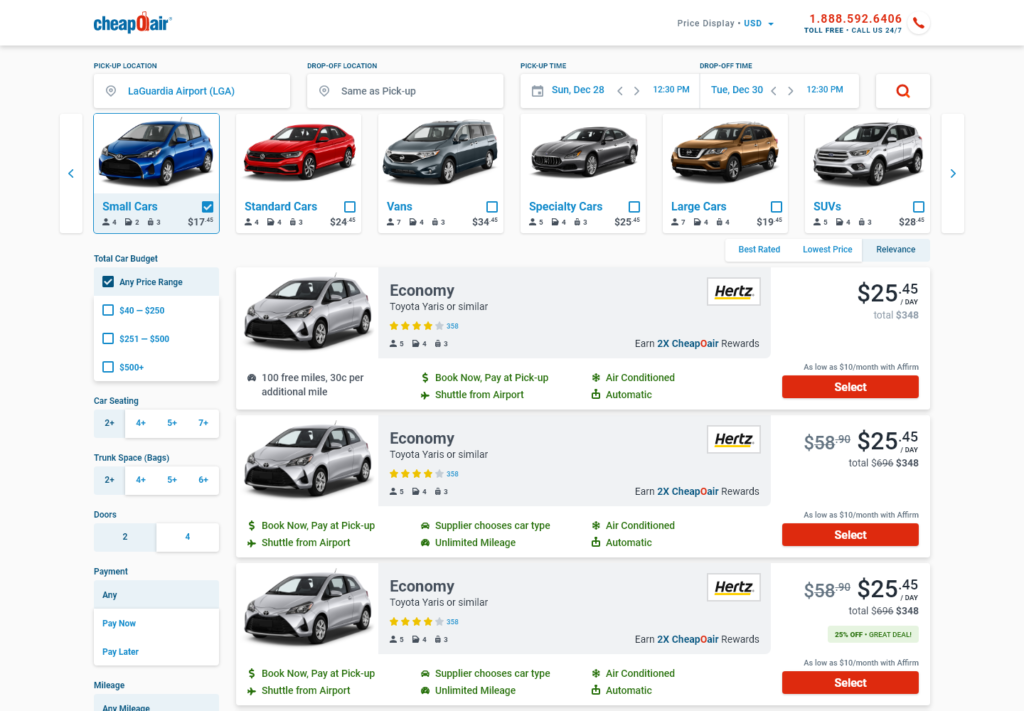At the top left corner of the image, there is a blue block-lettered text that reads "CHEAP". To the right of it, in red, are the characters "QOI" (though it is somewhat unclear). Continuing in blue letters, the text reads "AI." In the top right corner, there is a small gray symbol, either a registered trademark (®) or a trademark (™) symbol. 

Towards the right side of the screen, in small gray lettering, the text "Price Display" is shown alongside gray bullet points. Below this, there is another text in blue that reads "USD" in capital letters. A blue arrowhead pointing downwards indicates a drop-down menu option. 

Adjacent to this, a bold red phone number is displayed as "1.888.592.6406". Beneath the number, in small capitalized blue bold letters, it states "TOLL FREE" with a bullet point next to it and "Call us 24/7."

To the right of this information, there is a white circular icon with a shadowed gray border that features a red handset phone icon tilted to the left at the top. 

The bottom section of the image shows various car listings. On the left, there is an image of a blue car labeled "Small Cars" against a light blue background with a blue font. A blue tick box with a white check mark indicates selection, and directly beneath it, the price "$17.45" is shown in gray text.

To the right, there is an image of a red car labeled "Standard Cars" against a white background. Next to it is an unselected tick box, and beneath it, the price "$24.45" is displayed in gray text.